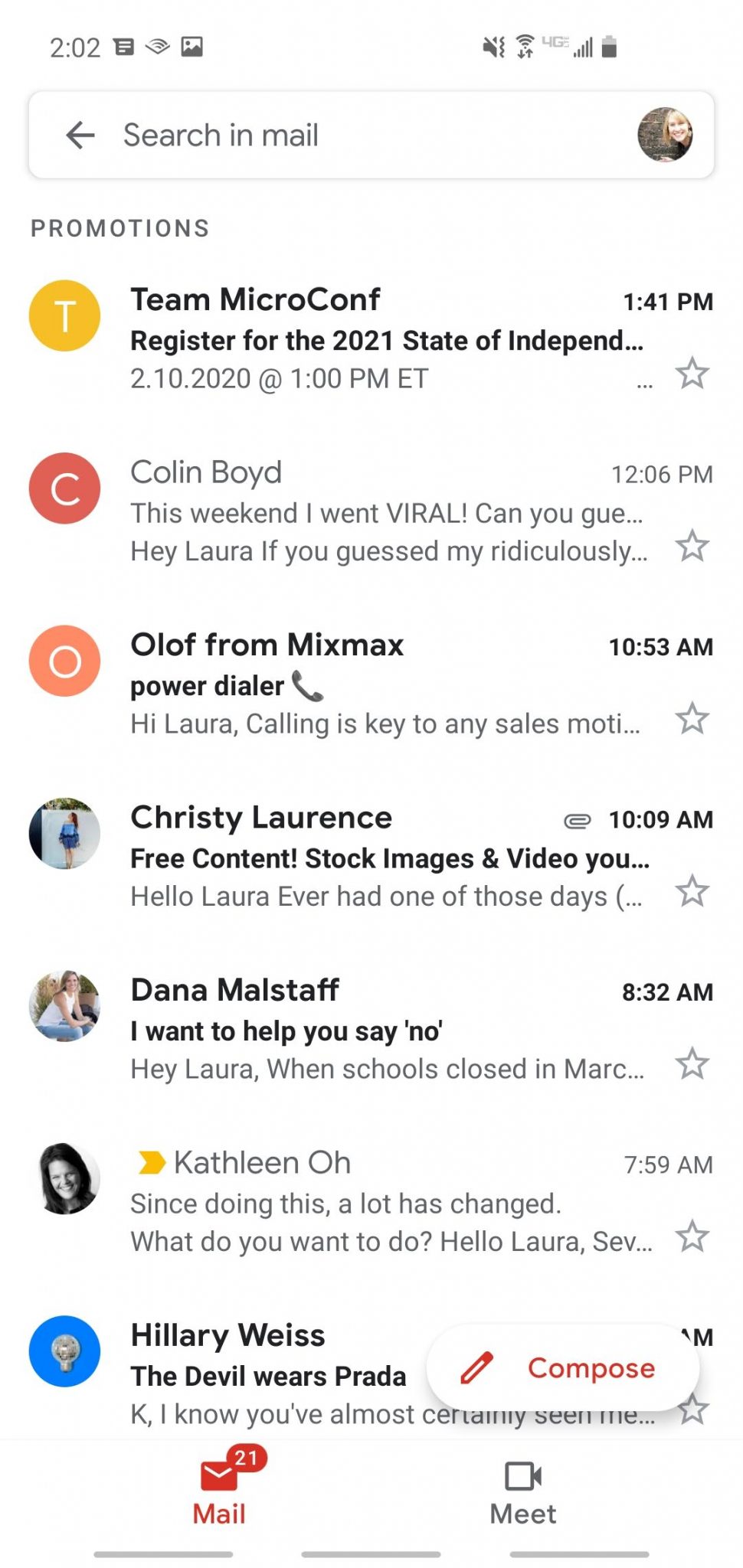A detailed screenshot of a phone screen is depicted, with the time reading 2:02 PM in the upper left corner. The top bar includes several icons: a messaging icon, a Wi-Fi symbol icon, a photo icon, a muted sound icon, another Wi-Fi icon, a Yu-Gi-Oh! icon, a phone signal icon, and a battery icon which is slightly above half full.

Below these icons, there is a prominent search bar, rectangular in shape. On the left side of the search bar, an arrow pointing left is visible, followed by the text "Search in Mail." On the far right side of this search bar, there is a circular profile picture of a white woman with blonde hair, set against a brick wall.

Underneath the search bar, the section labeled "PROMOTIONS" in all caps, features seven emails. The first email is from Team MicroComp with the subject "Register for 2021 State of Independent..." dated 2.10.2020 at 1:41 PM, marked with a yellow circle and a 'T' icon, and it’s unread. 

The second email from Colin Boyd with a red 'C' icon mentions "This weekend I went viral! Can you get...", received at 12:06 PM, is an unread message. 

The third email is from Olaf from Mixmax Power Dialer, signified with an orange 'O' icon. It has a subject line starting "Hi Laura, calling his key to any sales motivate..." and was received at 10:53 AM, and is unread.

The fourth email from Christy Lawrence has a subject "Free content! Stock images and video you..." with an attachment mentioned and is time-stamped at 10:09 AM. The icon for this email is a profile picture of a woman in front of a white wall, and the email is unread.

The fifth email, from Dana, with a subject "I want to help you say no. Hey Laura, when schools closed in March..." has an icon showing a white woman in a white tank top and blue jeans. It was received at 8:32 AM and remains unread.

The sixth email is from Catherine O., marked with a black-and-white headshot icon. The subject is "Since doing this, a lot has changed. What do you want to do?" and starts with "Hello Laura," received at 7:59 AM, and is read.

The final email, identified with a blue circle and a disco ball inside, starts with "The Devil Wears Prada, okay...". The time of receipt is partially visible with only 'AM' showing, and this message is also unread.

At the bottom of the screenshot, a red button labeled "Compose" is located, signifying the option to write a new email. The bottom bar shows "Mail" on the left side with 21 unread emails indicated in red text. On the right side of this bar is the "Meet" icon, labeled "Meet" in gray.